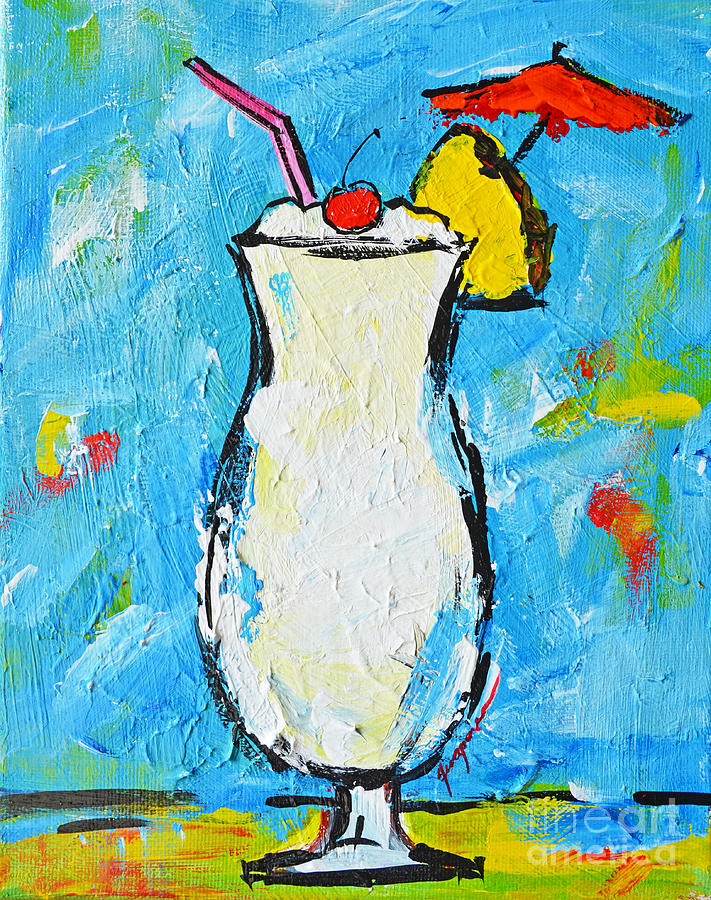The image depicts a detailed and vibrant hand-painted scene of a summery cocktail, possibly a piña colada or a vanilla milkshake, rendered in an oil painting style. The drink is housed in a teardrop-shaped, transparent glass outlined in black, filled with a creamy mixture of white and light yellow hues, suggesting a smooth beverage. A vivid pink straw extends from the left side of the glass, which is crowned with a small dollop of whipped cream and a bright red cherry at the top. Garnishing the drink, a slice of bright yellow pineapple sits on the rim, adorned with a tiny red cocktail umbrella. The background of the painting is a striking, vivid turquoise blue, dynamically interspersed with patches of white, yellow, red, and green brush strokes, invoking a lively sky. The surface beneath the glass combines greens, yellows, and reds, enhancing the summery and refreshing feel of the image. The painting bears a logo at the bottom that reads "The Art America" in transparent white text.